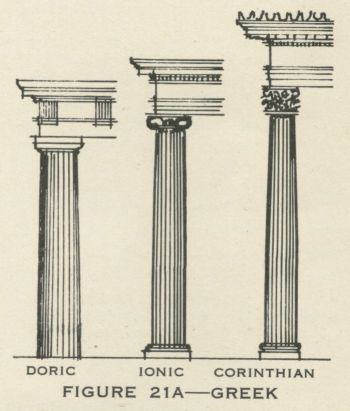This image is a detailed, hand-drawn, pen and ink illustration from what appears to be an architectural textbook, showcasing the differences between three styles of ancient Greek columns, arranged by height from left to right. The shortest column on the left is labeled Doric and is characterized by its plain, unadorned design and absence of a base stand. The middle column, labeled Ionic, is slightly taller, more ornate, and has a distinctive base at the bottom. The tallest column on the right, labeled Corinthian, is the most ornate, featuring intricate decorations and also includes a base. All three columns show numerous vertical lines running up and down their shafts, and at the top, the capitals display distinguishing stylistic elements that differentiate them. The illustration is captioned with "Figure 21a Greek" at the bottom, indicating its origin from a larger textbook or reference book on Greek architecture.